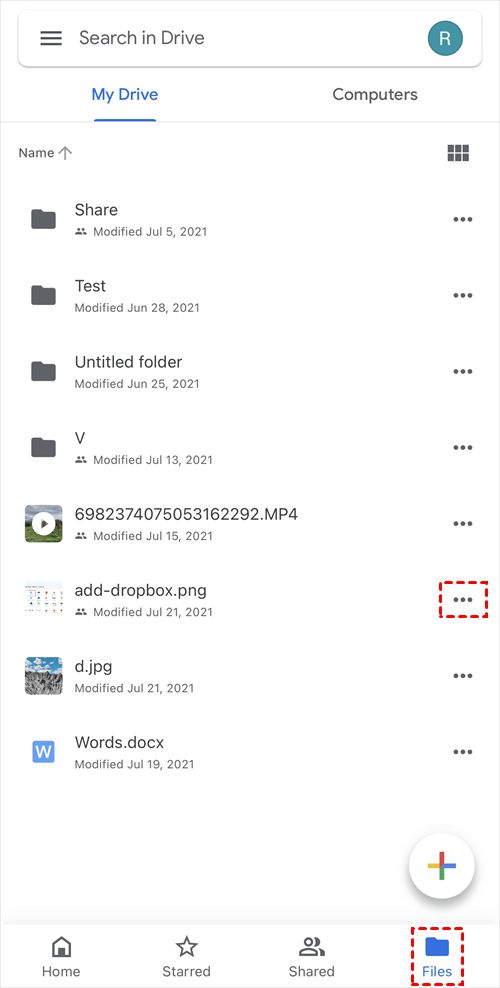This image is a mobile screenshot of a Google Drive session. The interface features a white background with a search bar at the top labeled ‘Search in Drive’, accompanied by three parallel lines (menu icon) to the left and a green circle with the letter ‘R’ inside it on the right. Below the search bar, there are two tabs: ‘My Drive’ and ‘Computers.’ The ‘My Drive’ tab is highlighted in blue and underlined, indicating it is currently selected.

The main content area displays a list of items within ‘My Drive’. The details of the items are as follows:

1. Folder named ‘Share’ - Last modified on July 5th, 2021.
2. Folder named ‘Test’ - Last modified on June 28th, 2021.
3. Folder named ‘Untitled Folder’ - Last modified on June 25th, 2021.
4. Folder named ‘V’ - Last modified on July 13th, 2021.
5. Video file named ‘6982374075053162292.mp4’ - Last modified on July 15th, 2021.
6. Image file named ‘add_Dropbox.png’ - Last modified on July 21st, 2021.
7. Image file named ‘D.jpeg’ - Last modified on July 21st, 2021.
8. Word document named ‘words.docx’ - Last modified on July 19th, 2021.

At the bottom of the screenshot, there are four navigation options: ‘Home’, ‘Starred’, ‘Shared’, and ‘Files’. The ‘Files’ option is selected and highlighted in blue. Additionally, there is a red dotted line box around the entire area.